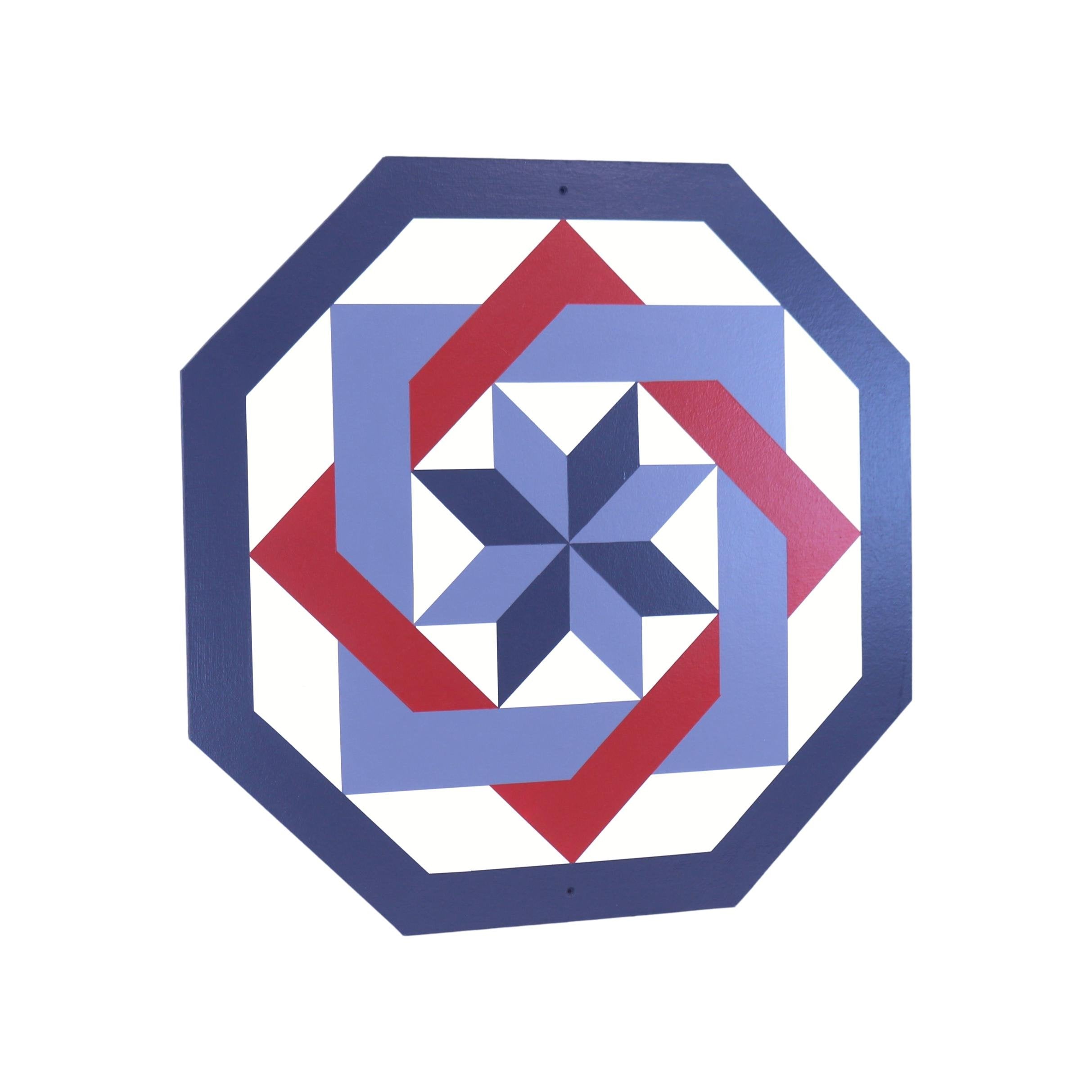The image features a central design set against a white background with no text or outer border. The main shape is a large octagon with a thick dark bluish gray border. Nested within this octagon is a red diamond shape, which has a thick border and intersects with a lighter blue square, creating a hugging effect. At the very center of this diamond and square intersection, there is an intricate star shape created by eight alternating light blue and dark blue trapezoids. This star forms another smaller octagonal shape at its core. The overall composition consists of the outermost octagon, followed by the red diamond and blue square entangled within it, and a two-toned star at the center made up of eight trapezoids.